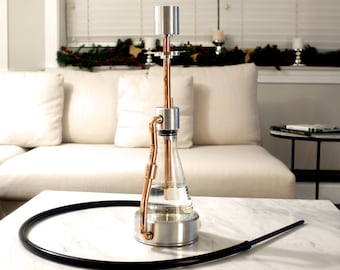In this color photograph, framed in landscape orientation, the focal point is a modern-styled hookah placed prominently on a sleek, white marble table with gray veins. The hookah features a glass beaker-shaped base with aluminum and copper fittings on top and a brass handle on its left side. A black hose, attached to the back of the hookah, coils elegantly across the table, leading to a nozzle on the right.

The setting is a contemporary, minimalistic living space. Directly behind the table is a modern, armless white sofa adorned with throw pillows. An end table, small and black, sits adjacent to the sofa, holding a stack of books. Further back, a windowsill spans the width of the scene, lined with green plants and several white candles perched on silver stands. The blinds behind the windowsill are closed, adding to the cozy and intimate atmosphere captured in this realistic representation.